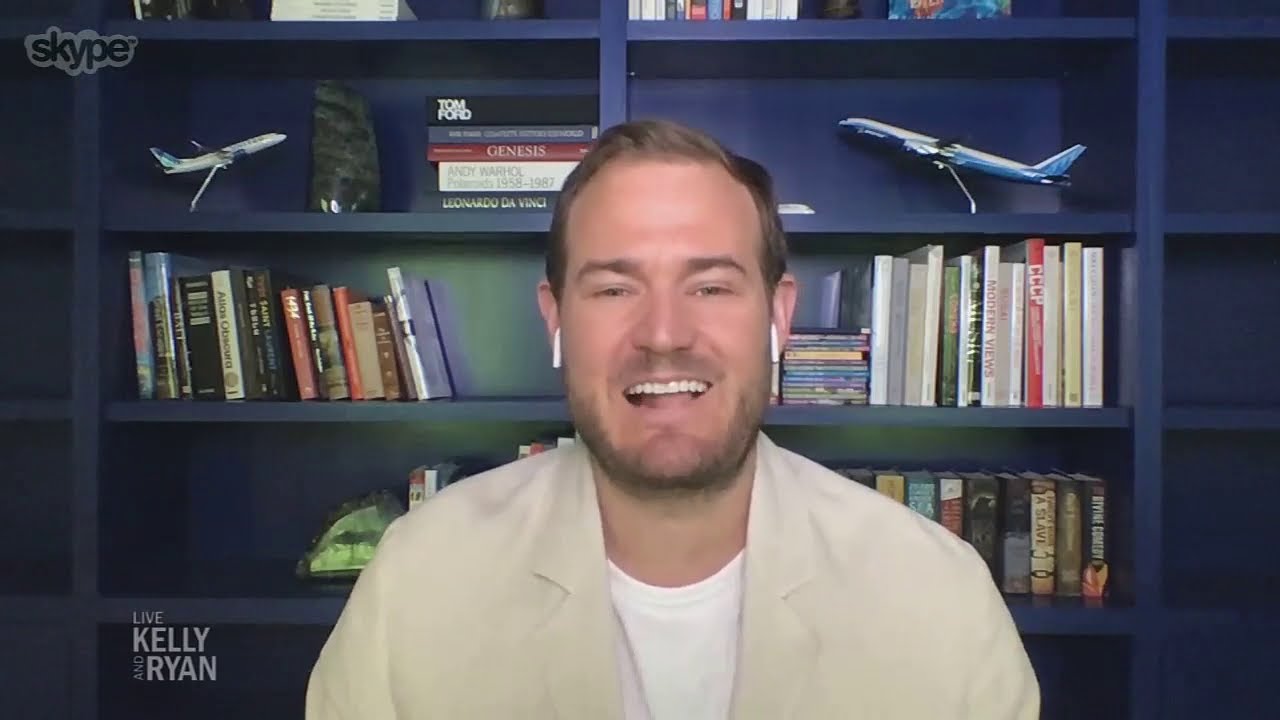A man with light to medium brown hair, styled short, sits in front of a large blue shelving unit. He is wearing a tan jacket over a white t-shirt, and has a short stubble beard and mustache, complemented by strong eyebrows. White Apple AirPods are visible in his ears. He has a light, engaging smile on his face, as if mid-conversation, with his mouth slightly open showing his teeth. The shelving unit behind him is filled with various items including books, model airplanes, and a shiny marble rock placed between some books. The background prominently displays text in white; "Nye" and "Live Kelly and Ryan" are situated on the lower left, as well as "Skype" in the upper left corner, suggesting a live televised or streamed interview. In the upper left corner, a graphic of a skateboarder is also visible.